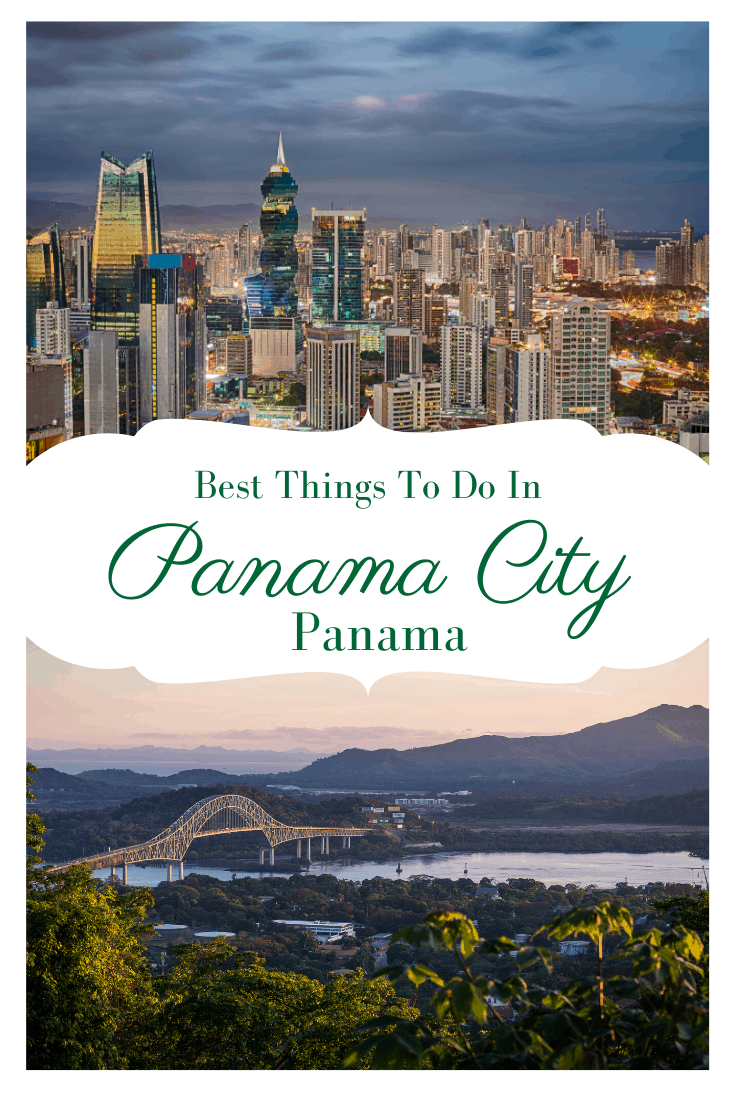A breathtaking scene showcases a majestic bridge spanning a tranquil body of water, with the backdrop of a sprawling cityscape and distant, rugged mountains. The foreground is rich with greenery, including a variety of lush trees and elegant palm trees, all illuminated by the soft, warm hues of what appears to be a sunset. The sky is painted with the delicate, golden light of the setting sun, lending a serene and romantic ambiance to the scene. At the center of the image, a white circular emblem prominently displays the words "Best Things to Do in Panama City" in green text, with "Panama City" elegantly written in cursive, while the rest of the text remains in a standard font. This picturesque portrait beautifully captures the essence and allure of Panama City.